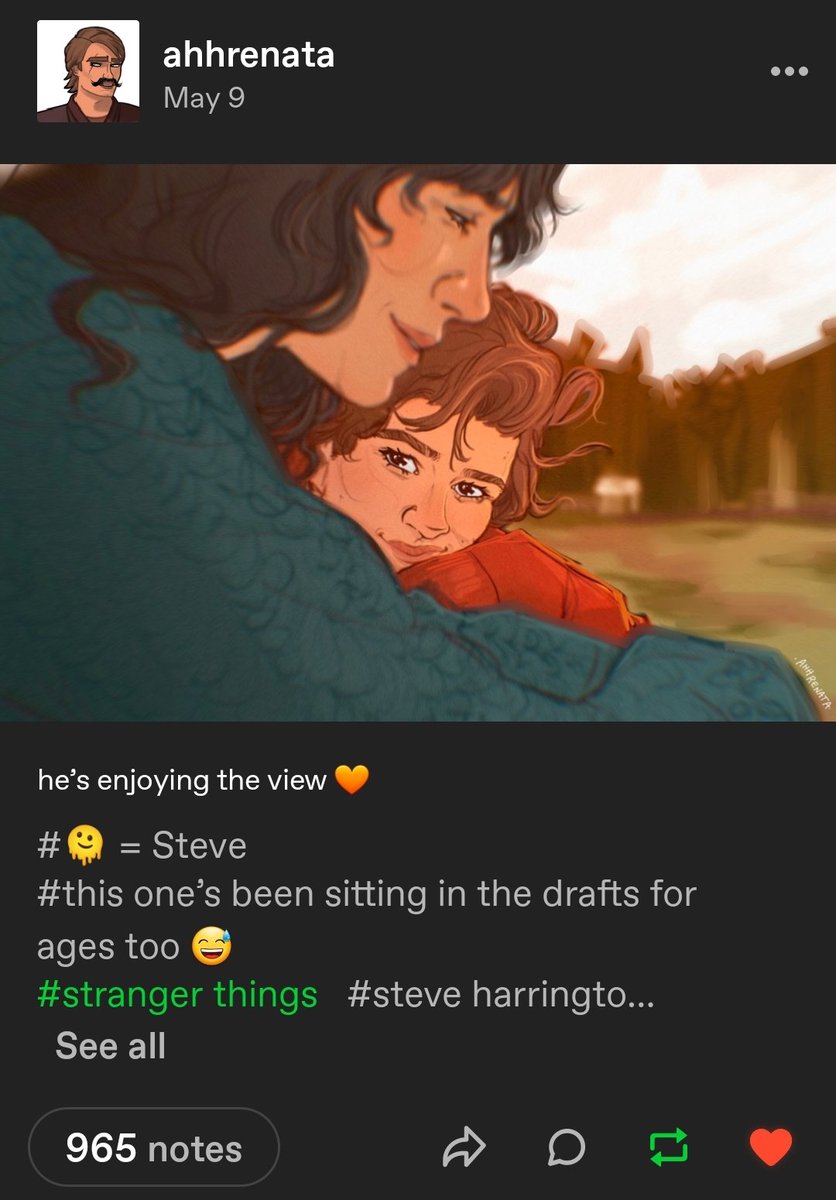In this vibrant illustration, Renata captures a scene featuring a man with a mustache and short brown hair. The image is marked with a timestamp of May 9th, and three dots to the right indicate the presence of a cartoon drawing. The drawing portrays two women seated next to each other; one is wearing a blue long-sleeved shirt, while the other dons a red shirt. They appear relaxed and content against a backdrop of lush trees and greenery. The man, seemingly named Steve, appears to be enjoying the scenic view. This piece has been tagged with several hashtags, including #Steve, #ThisOnesBeenSittingInTheDraftsForAges, #StrangerThings, and #SteveHarrington. The post has garnered 965 notes, represented by an arrow, a comment symbol, two green circling arrows, and a red heart emoji.